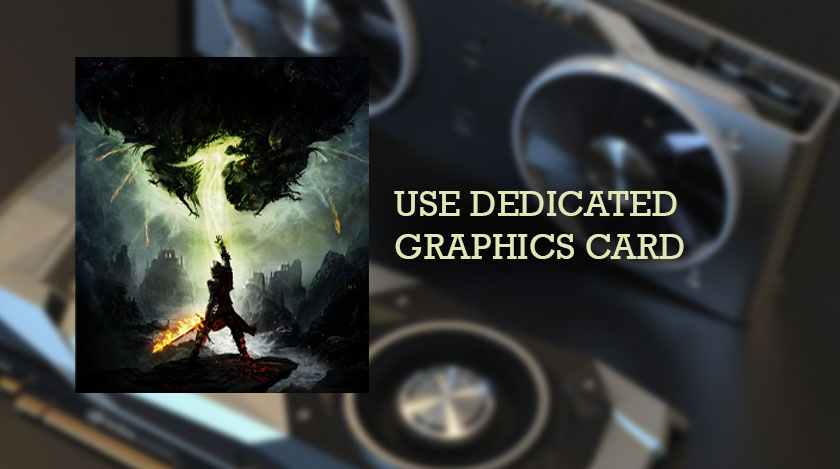The rectangular image, significantly wider than it is tall, appears to be a poster for an album with a dramatic and gothic theme. Prominently displayed in pale yellow letters slightly to the right of the center, the text reads "USE DEDICATED GRAPHICS CARD." The background features a blurry image of what seems to be two boom boxes or another type of electronic device with multiple circular components, possibly speakers, angled and arranged in a complex pattern.

To the left of the text is a striking square album cover. It depicts a gothic scene with a man standing dramatically amidst ominous surroundings. The man, a dark silhouette, is raising his right arm towards the sky, from which jagged, lightning-like yellow light emanates. He appears to be holding a flaming sword with his legs set wide apart. The backdrop includes dark clouds, shadowy mountains, gray buildings or rocks, and a stream. Beneath him, fire glows at his feet. Above, fireworks-like sparks of yellow light burst from the black clouds, creating an intense, visually arresting scene that draws the viewer's eye. The overall dark, dramatic atmosphere of this composition complements the eerie and powerful nature of the album's theme.